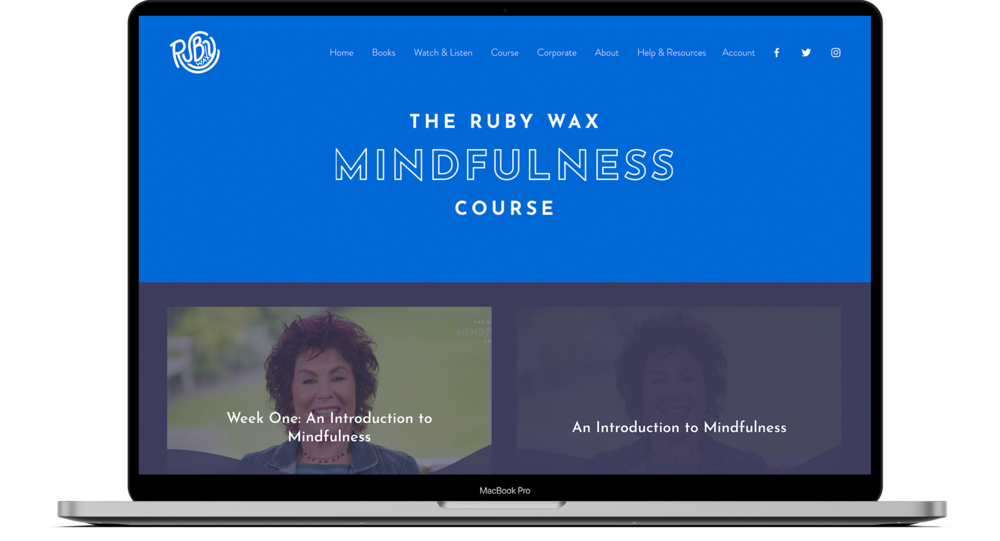In this detailed image, an open MacBook Pro is prominently displayed. The laptop screen features a black rim around the edges, with the recognizable silver casing of the MacBook Pro visible at the bottom. The top half of the screen is light blue, displaying a white logo with the letters "RB" arranged in a circular shape. A taskbar stretches across the top of the screen, listing various navigation options: Home, Books, Watch and Listen, Course, Corporate, About, Help and Resources, and Account. Social media icons for Facebook, Twitter, and Instagram, all in blue, are positioned to the far right of the taskbar.

Directly below this, the name "Ruby Wax" is prominently displayed in bold white print. Beneath her name, the text "Mindfulness Course" is featured, with the word "mindfulness" highlighted in blue. This text collectively reads as "The Ruby Wax Mindfulness Course."

Further down, two images of an older Caucasian woman with short, reddish hair are displayed side-by-side. The woman is set against a green background in both images. The image on the left is clear and labeled "Week One: An Introduction to Mindfulness." The image on the right, however, is darkened, with the same label, "An Introduction to Mindfulness," suggesting it’s the same image as the left one but with a shaded or tinted effect.